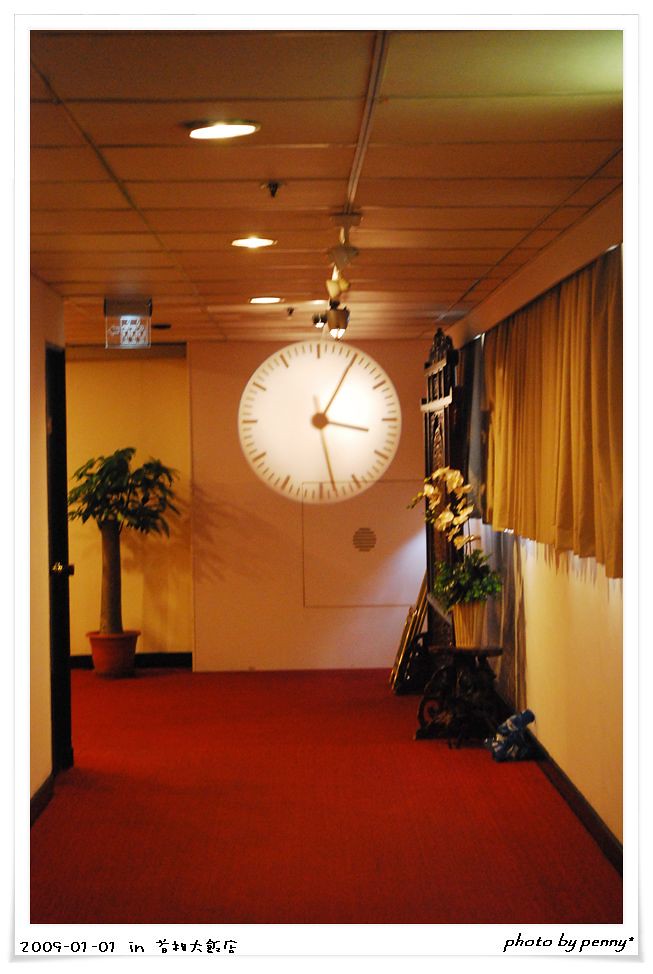This photo captures a dimly lit hallway with a red carpet. The walls are an orangish yellow, possibly due to the low lighting conditions. On the right side, thick curtains partially drawn over a window let in a sliver of natural light. Just beyond the curtains, a tall structure, resembling a pagoda adorned with flowers, reaches from floor to ceiling. Straight ahead, the ceiling is lined with lights, and a large clock projection dominates half of the end wall, showing the time as approximately 3:05, likely in the afternoon. To the left, there is a decorative fake tree and a plant nearby, leading up to a door marked by an exit sign.